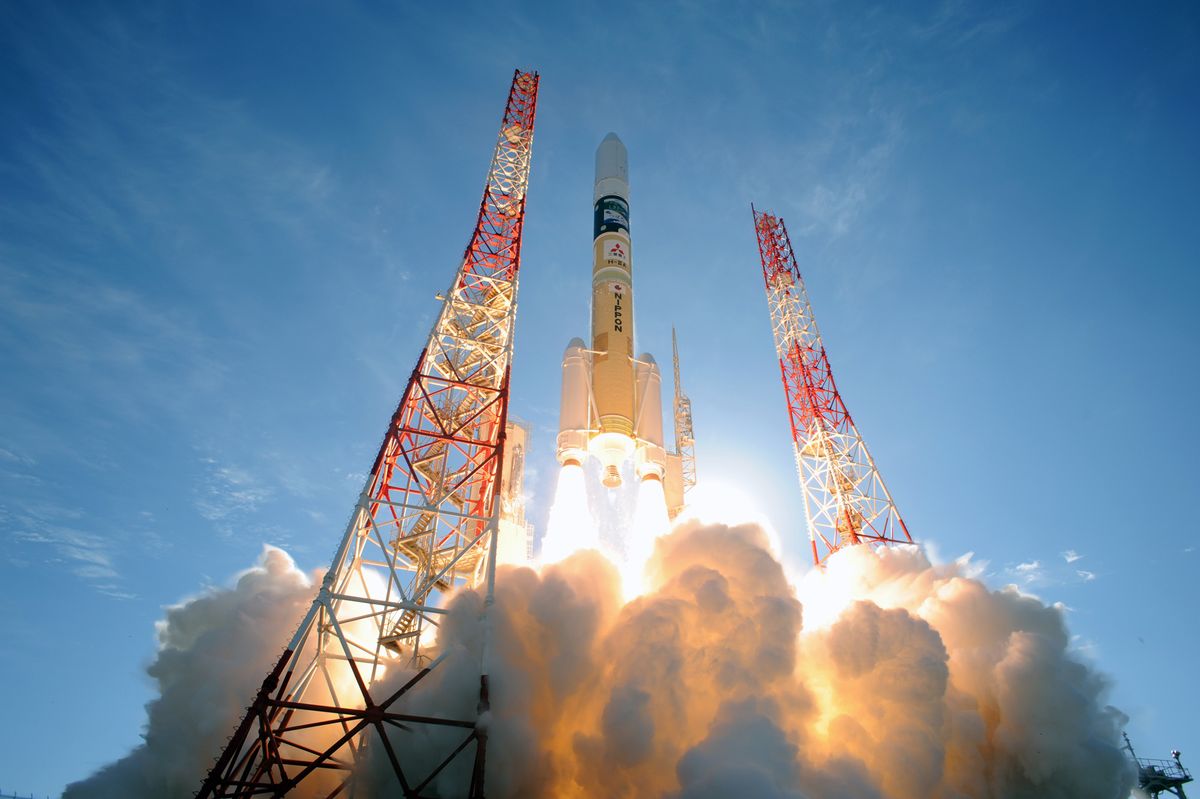The photograph captures the dramatic launch of a rocket soaring into a clear, bright blue sky dotted with a few wisps of clouds. The rocket is bathed in flames as it propels upward, leaving behind billowy plumes of smoke and exhaust. The rocket itself is tall and slender with a cream-colored body that transitions to dark hues near the top, ending in a white tip. It is flanked on either side by towering red and white scaffolding that once stabilized it. The lower section of the rocket emits bright yellow flames, adding to the spectacle. Despite the varying descriptions of colors on the rocket, its journey skyward is a breathtaking marvel of engineering amidst a day with perfect weather, signifying the commencement of its space mission.